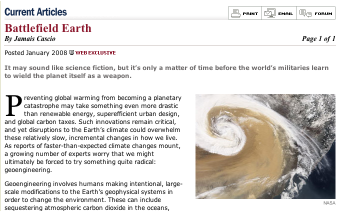The image displays an article layout with the following details: 

- **Top Left Corner:** The text "Current Articles" is prominently featured in blue.
- **Top Right Corner:** Three functional buttons labeled "Print", "Email", and "Forum" are written in black and provide user interaction options.
- **Left Side Below "Current Articles":** There is a heading "Battlefield Health" in black. Right below it, the article is attributed to JAMA, posted in January 2018.
- **Article Body:** The main text of the article is written in black against a white background. Although blurred, the visible excerpt discusses the potential use of geoengineering by militaries to combat climate change. It emphasizes the urgency of addressing global warming, suggesting that even innovative designs and carbon taxes might not be sufficient. The topic of geoengineering, which involves intentional large-scale modifications of Earth's geophysical systems, is highlighted as a radical yet necessary measure.
- **Image on the Right Side:** There is a picture of a cyclone, depicted with white, brown, and gray colors.